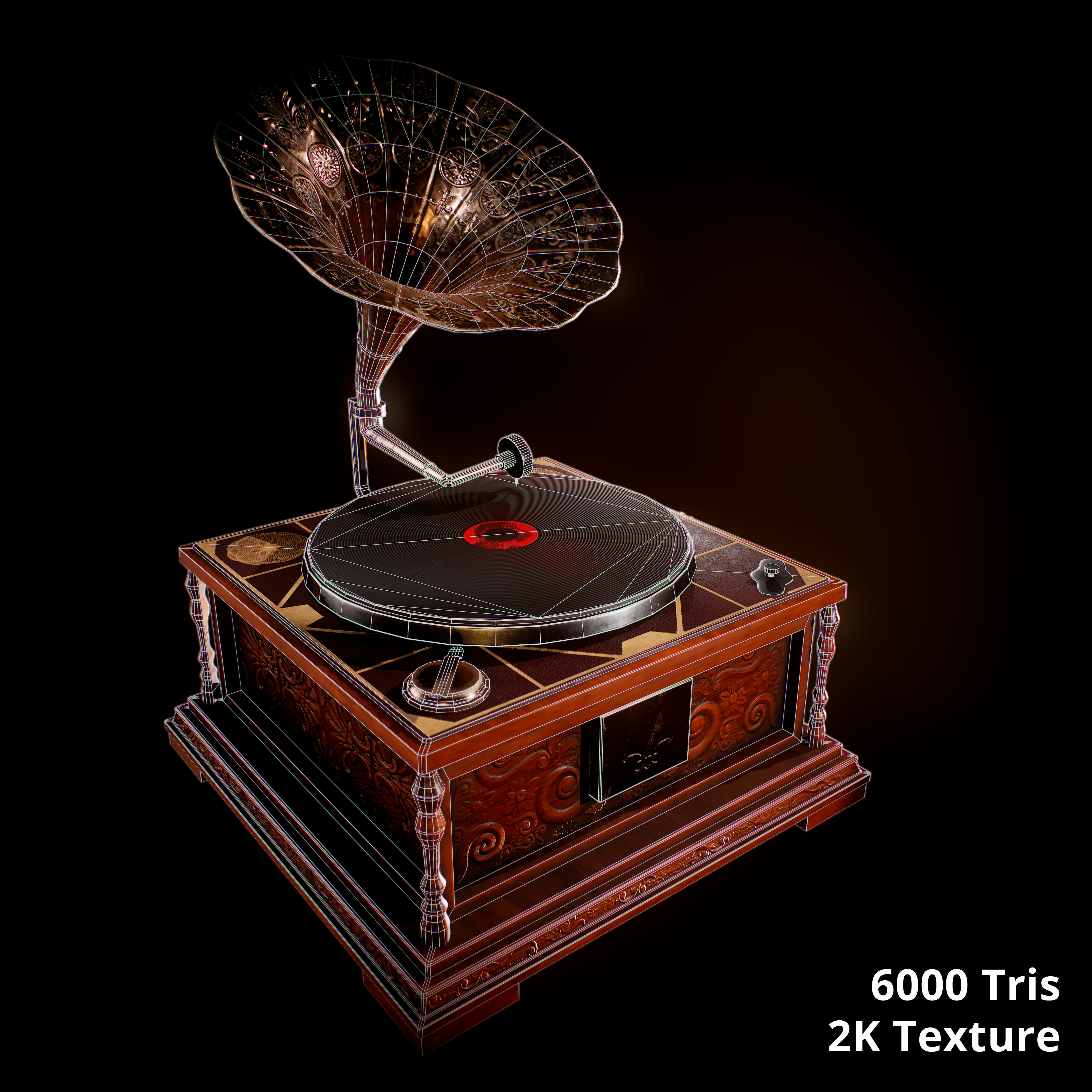The image depicts a highly detailed, computer-generated phonograph set against a completely black background. The phonograph has a square, dark-stained wooden base adorned with intricate scroll patterns on all four sides and a gold geometric design on the top surface. The center of the record-playing area is bright red, adding a striking contrast. Emerging from the top is an ornate, flute-like horn speaker, distinguished by its bronze or darker metallic finish and embellished with a pattern of circles and scroll lines. The horn, which appears very elaborate and fancy, suggests a blend of vintage aesthetics and modern design. In the bottom corner of the image, there is a white inscription that reads "6000 TRIS 2K Texture."